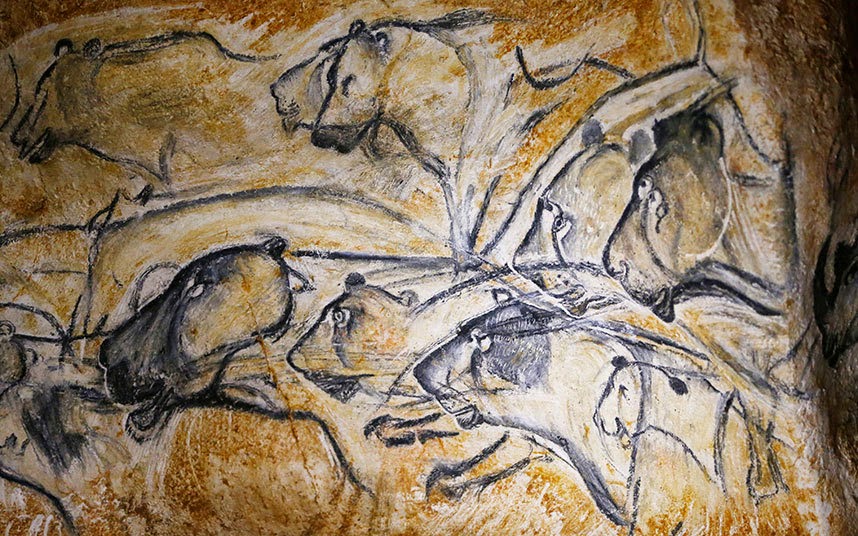This image features a detailed, modern interpretation of cave paintings displayed on an orangey-yellow surface, possibly mimicking rock or leather. The focal point is a series of intricately sketched animal heads, resembling big cats such as cheetahs, leopards, or bears, rendered mainly in charcoal or ink. The drawings are organized into two rows; the animals on the bottom row appear larger and more detailed than those on the top row. The heads are outlined with precision, highlighting features like the jaws, eyes, and ears, but their necks fade into the background, creating a splotchy, overlapping effect. Some areas show black or dark blue shading, adding depth and contrast against the lighter, chiseled or worn away portions of the background. A subtle black shadow is present to the right, adding to the dimensionality of the piece. Overall, the artwork captures the essence of ancient cave art while presenting it in a contemporary style.